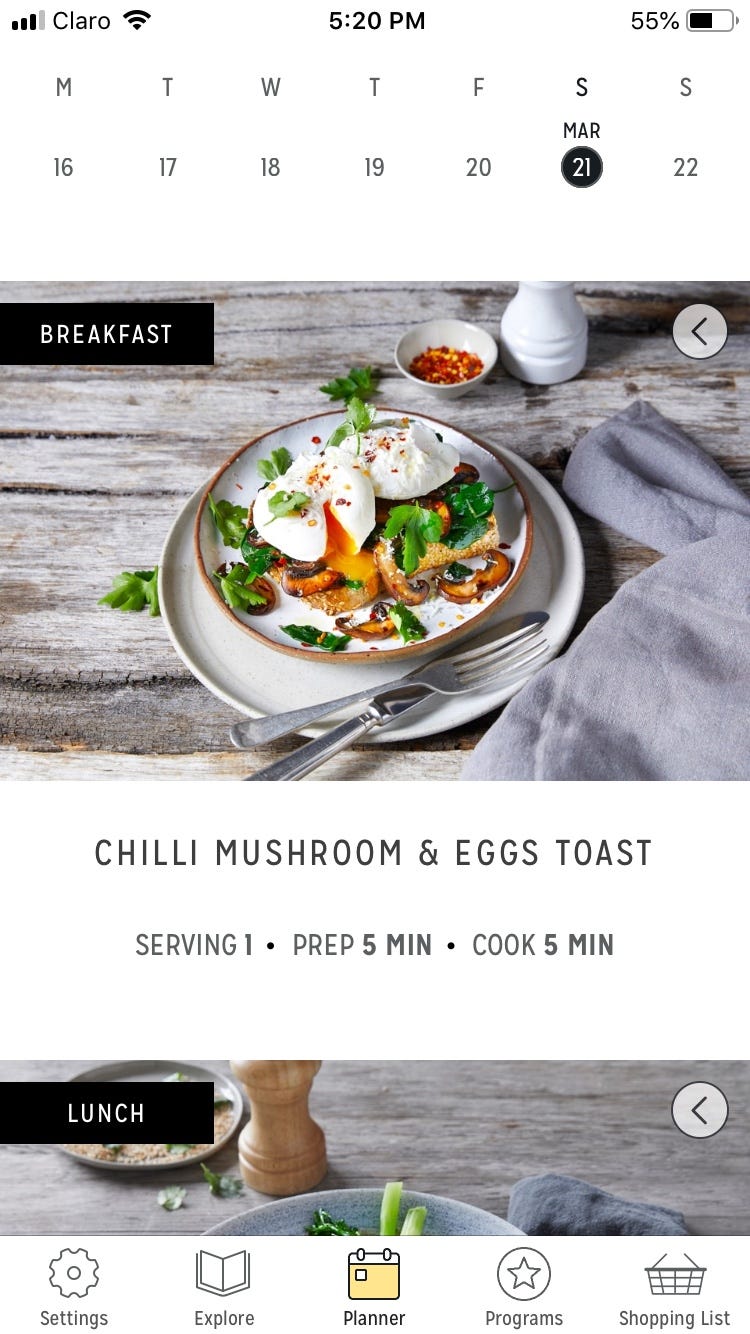The image appears to be a detailed screenshot from a mobile device, displayed in a vertical, rectangular format. At the top of the screen, the status bar is visible, showing the Wi-Fi signal indicator on the left, the current time centered, and the battery symbol indicating 55% on the right.

Below the status bar, there is a section that appears to be part of a calendar interface. The days of the week are listed horizontally as "MTWTFS", representing Monday through Sunday. The date "Saturday, March 21st" is highlighted, indicating it is currently selected.

Directly beneath the calendar, a detailed meal planner is visible. The word "Breakfast" is prominently displayed in a black box located in the upper left corner of this section. An image showcases a plate with a bowl on top, containing a meal that includes mushrooms, toast, eggs, and assorted vegetables. Silverware is positioned next to the plate. The description underneath reads, "Chili, mushroom, and eggs toast - Serving: one, Prep time: 5 minutes, Cook time: 5 minutes."

Further down, a smaller rectangle is labeled "Lunch." Only part of this meal section is visible at the bottom of the image, showing a plate with green vegetables, a salt or pepper shaker (possibly a pepper grinder), and an additional plate partially in view on the upper left.

At the very bottom of the screenshot, a navigation bar displays several icons: Settings, Explore, Planner, Programs, and Shopping List. The "Planner" icon is highlighted in yellow, indicating it is the currently selected menu.

This image captures an organized presentation of daily meal planning on a mobile application interface.